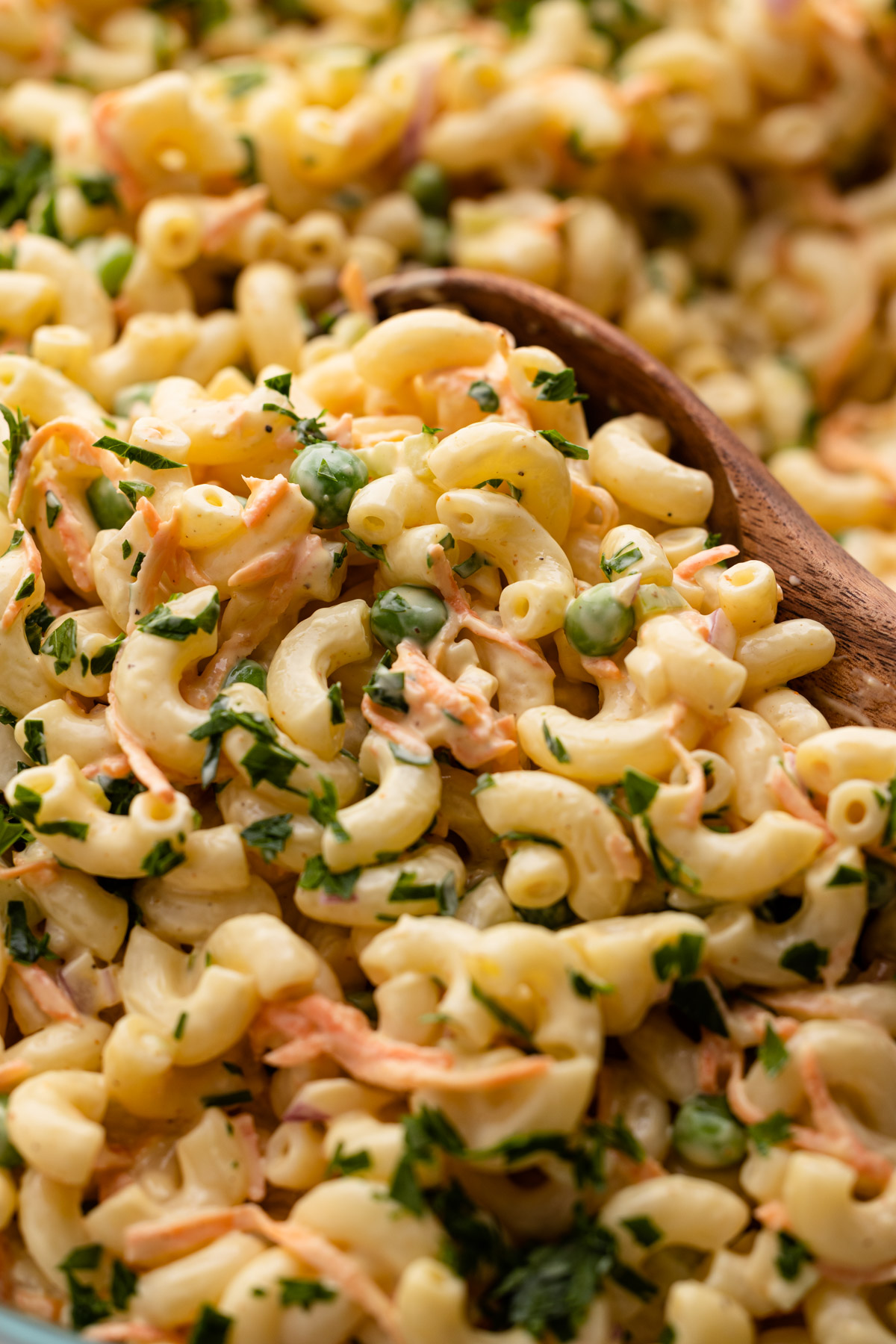This high-quality, close-up image showcases a delectable macaroni and cheese dish. The pasta, likely small elbow macaroni, is bathed in a creamy, yellow sauce, which is not overly goopy. There are flecks of green herbs and small, shredded orange bits, possibly carrots or crab, intermixed with the pasta. The grains cling to the macaroni, adding texture to the dish. A flat wooden spoon can be seen partially submerged under the pasta, poised to scoop a portion. The foreground macaronis are in sharp focus, while the background macaronis are artfully blurred. Light softly illuminates the dish, enhancing its appetizing appearance. In the bottom left corner, a peculiar metallic object is faintly visible.